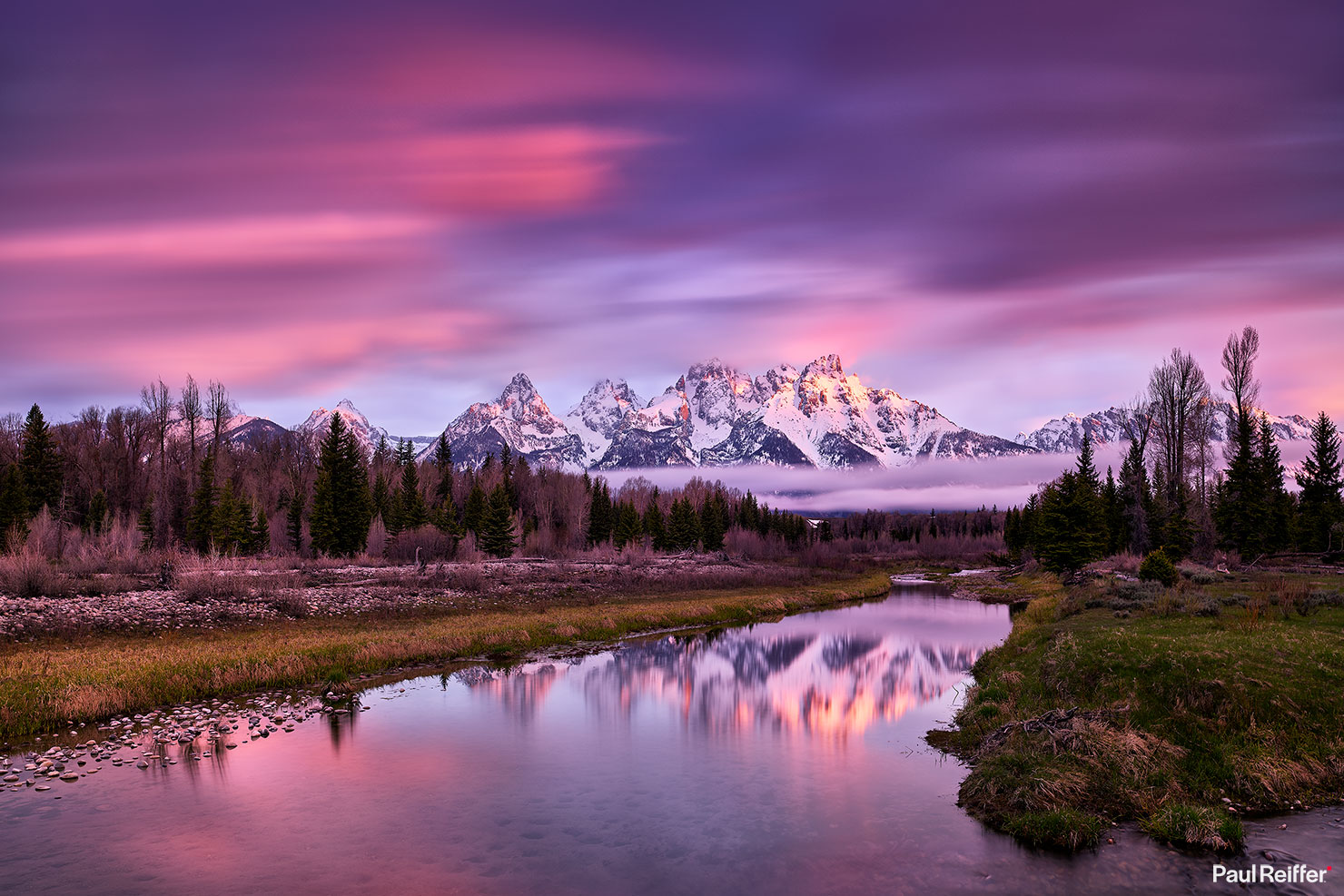This image captures a breathtaking outdoor scene, possibly taken during sunrise or sunset. The vibrant sky is adorned with shades of purple and fuchsia pink, creating a striking backdrop for the landscape. Dominating the background is a snow-capped mountain range, with various shades of dark gray rock adding texture to its rugged appearance. At the base of the mountains, wisps of thin clouds settle gently.

In the foreground, a serene creek or small river winds through the center of the image, its glassy surface reflecting the majestic mountains and colorful sky above. On the left-hand bank, a dense forest of pine trees and barren brown trees stands tall, interspersed with patches of both lush green and dried grass. Big rocks add a rustic charm to this side of the creek. The right-hand bank mirrors the left, featuring additional trees and a grassy area that enhances the natural beauty of the scene.

The image also features delicate details such as the shoreline on either side of the creek and a signature "Paul Reifer" in white lettering at the bottom right-hand corner, marking the artist's work. This panoramic view not only showcases the harmony between the elements of nature but also captures the silence and tranquility of this beautiful moment in time.